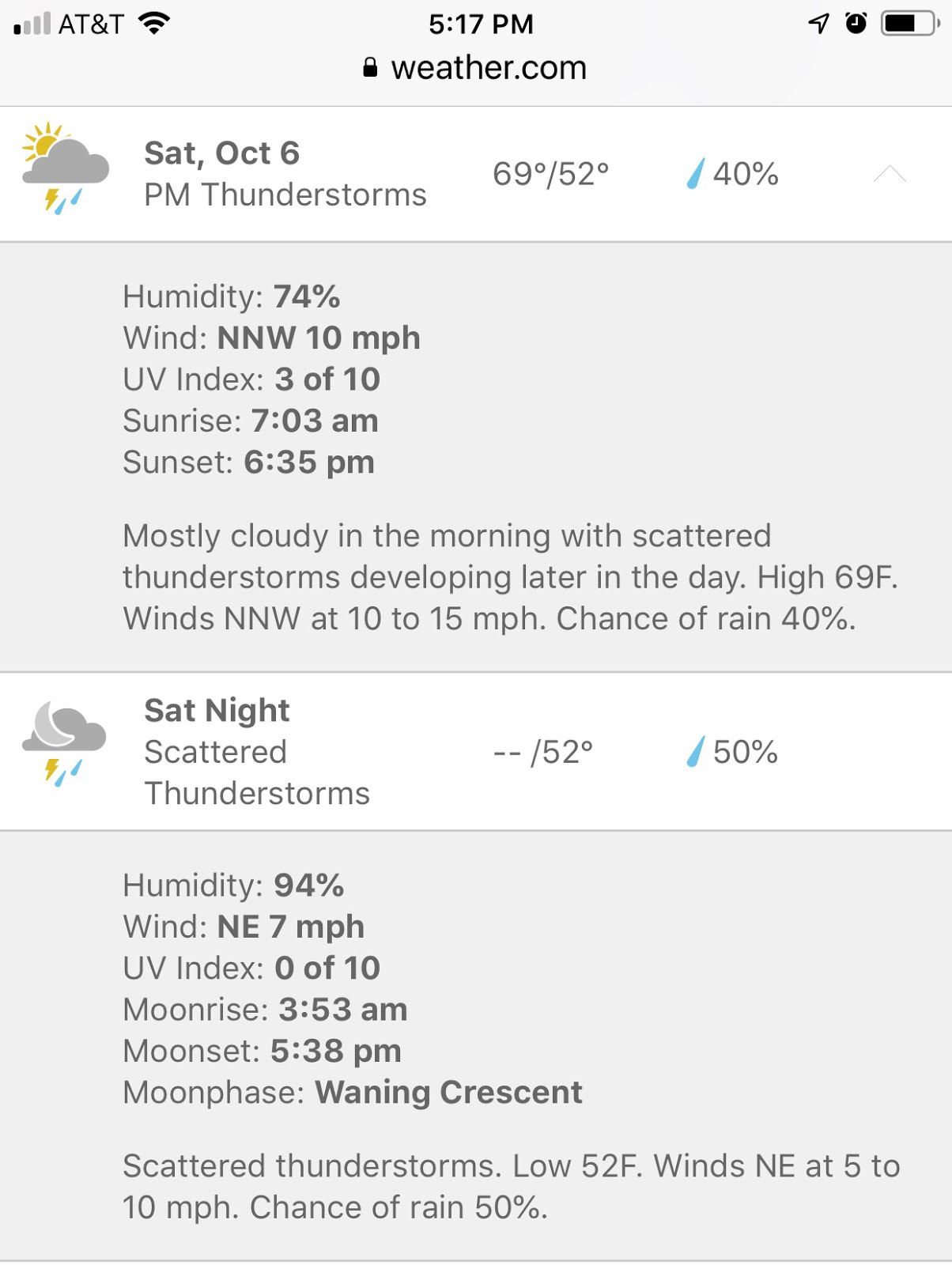This image is a detailed smartphone screenshot taken at the top left corner of the display. The device is connected to AT&T with one signal bar and a full Wi-Fi symbol. The time displayed is 5:17 PM, and there is a lock icon shown next to the web address weather.com. The battery icon indicates approximately three quarters of a charge remaining.

On a white background, the weather forecast is prominently displayed. A graphic shows a sun partially obscured by a cloud, along with a lightning bolt and rain, symbolizing a thunderstorm. The forecast reads: "Saturday, October 6th PM, Thunderstorm, 69°F / 52°F." It also mentions a 40% chance of rain.

Further details are provided in a light gray box beneath the main forecast: 

- Humidity: 74%
- Wind: North-Northwest at 10 MPH
- UV Index: 3 out of 10
- Sunrise: 7:03 AM
- Sunset: 6:35 PM

Below this box, an additional weather summary states: "Mostly cloudy in the morning with scattered thunderstorms developing later in the day. High 69°F. Wind: North-Northwest at 10 to 15 MPH. Chance of rain: 40%." 

This comprehensive screenshot gives a full overview of the expected weather conditions, alongside specific details like humidity levels, wind speed and direction, along with UV index, sunrise, and sunset times.